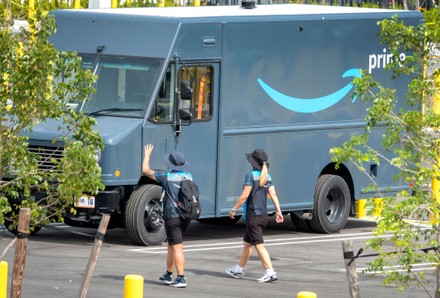In the center of the image, a large, boxy, dark blue-gray Amazon Prime delivery truck is partially obscured by trees, their branches framing the scene on both the left and right. The truck prominently features a turquoise Amazon arrow logo pointing to the word "Prime" in white text. The truck is parked in an otherwise empty parking lot. Positioned at the bottom of the image are several yellow poles and sticks supporting the trees, directing traffic within the lot.

Two Amazon workers are walking towards the delivery truck, which is glimpsed from the driver's side, partially obscured by the workers themselves. The person on the left, wearing a dark blue hat and a dark blue and teal Amazon-branded shirt with a white arrow logo, has a black backpack on and is lifting their left arm, possibly waving. They are also dressed in black knee-length shorts, bluish tennis shoes with white soles, and black socks. The person on the right features long blonde hair peeking out from under a black visor hat. They are wearing an identical Amazon shirt, black shorts, white tennis shoes, and white socks.

The background includes a few unidentifiable elements, but the focus remains on the depicted Amazon Prime delivery truck and its approaching workers.